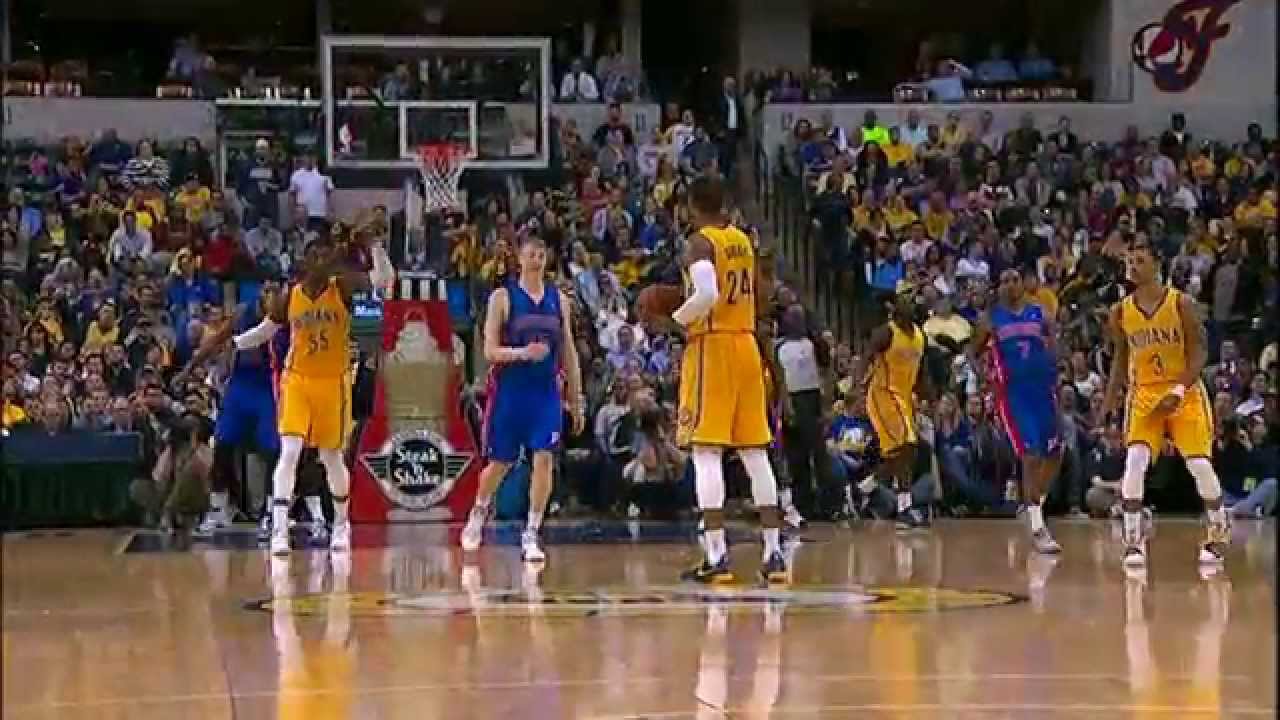The image depicts a nostalgic, possibly 1990s, basketball game taken from the side of the court. In the center, a player in a yellow uniform, labeled "Indiana," holds the ball. To his left and in front of him, a blue-uniformed player stands, with another yellow-uniformed player beside him and a blue-uniformed player behind. The orange-rimmed, clear backboard basketball hoop is visible in the top left corner, indicating their close proximity to the basket. The court is a well-polished, light brown hardwood with an indistinct emblem at its center. Spectators fill the stands in the background of this smaller, intimate venue, possibly hinting at a college or international game. The players appear to be in a moment of pause, perhaps strategizing or socializing before the game resumes. The image quality is low, characteristic of older photography technology, adding to its vintage charm.